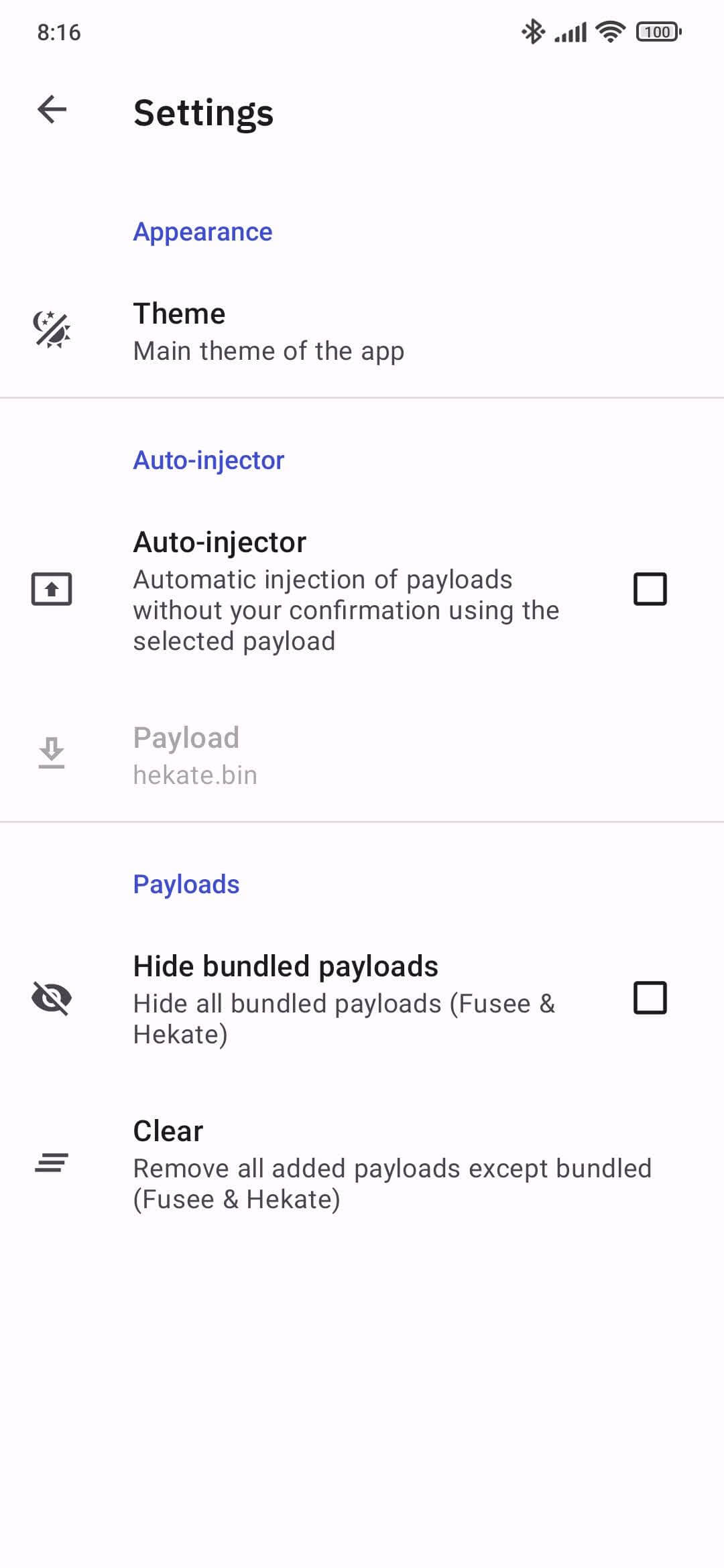**Screenshot of a Mobile Settings Page**

The image is a screenshot of a mobile device's settings page with a white background. 

- **Header Information:**
  - In the top left corner, the time is displayed as "8:16".
  - The top right corner features three icons:
    - A diamond-shaped grid or checkerboard.
    - A cell signal strength indicator with five ascending bars.
    - A full Wi-Fi signal icon.
    - A battery icon displaying "100", indicating full charge.

- **Main Content:**
  - Beneath the top icons, there is a left-facing arrow and the bold text "Settings".
  - Below the "Settings" label, the blue text "Appearance" is shown.

- **Settings Options:**
  - **Theme:**
    - Depicted with an icon of a moon, a diagonal line, and a sun in black and white.
    - To the right, it reads "Theme" with the description "Main theme of the app".
    - This section is separated by a thin horizontal gray line.
  
  - **Auto Injector:**
    - Highlighted with blue text "Auto Injector".
    - Accompanied by an icon of a rectangle with an upward-facing arrow.
    - To the right, it reads "Auto Injector" with the description: "Auto injection of payloads without your confirmation using the selected payload".
    - Next to this description is an unchecked open box.
    - Below this is grayed-out text "payload hectate.bin" with a corresponding grayed-out icon of a downward-facing open arrow pointing to a small horizontal gray line.

- **Additional Options:**
  - Separated by another thin horizontal gray line.
  - **Payloads:**
    - Marked with blue text "Payloads".
    - Includes an icon of an eye with a diagonal line through it, indicating "hide".
    - Next to this is the text "Hide Bundled Payloads" and the description "Hide all bundled payloads (FUSI and hectate)". An adjacent unchecked open box is presented.
  
  - **Clear:**
    - An icon with three slightly angled horizontal lines, where the top line is more to the right of the bottom line.
    - Next to this, it reads "Clear" with the description: "Remove all added payloads except the bundled payload (FUSI and hectate)".

This detailed description captures all elements and their layout on the mobile settings page, providing a comprehensive overview.